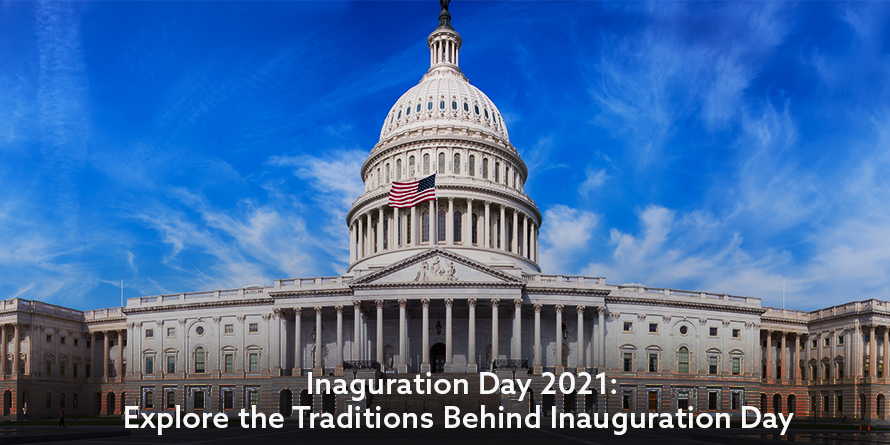This is a wide-angle photograph taken during the day of the U.S. Capitol building in Washington, D.C. The image beautifully captures the iconic structure from the front, showcasing its gray stone facade and distinctive domed top, some parts of which are slightly faded to red. Above the columned portico, the American flag is visibly blowing from right to left against a backdrop of a clear blue sky adorned with wispy white cirrus clouds. At the bottom of the photograph, white sans serif text overlays the scene, reading, "Inauguration Day 2021: Explore the Traditions Behind Inauguration Day." Notably, "Inauguration" is misspelled as "NAGURATION" in the first instance. The photograph emphasizes the building's grandeur and the solemnity of the event it references, with no people present to distract from the architectural beauty and the serene atmosphere.